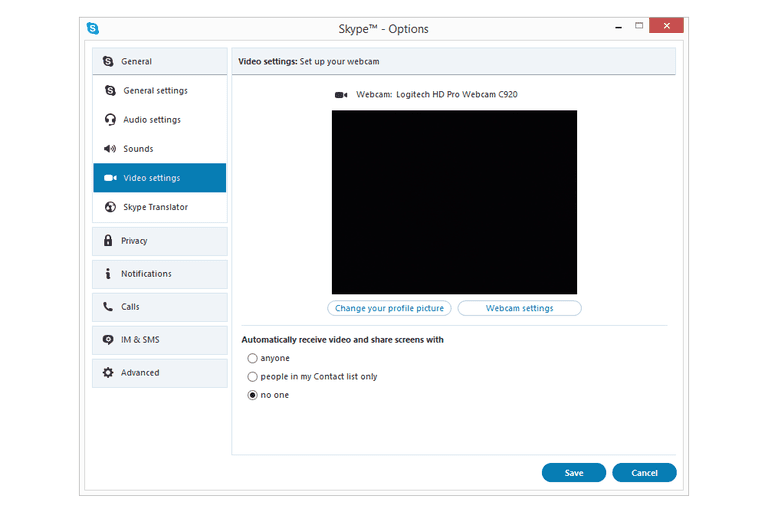A detailed description of a Skype video conferencing options webpage, showcasing the interface and settings:

The displayed webpage is a settings page for Skype's video conferencing features. At the very top, the iconic "Skype™" logo is prominently visible, accompanied by typical window control buttons for minimizing, resizing, and closing the window.

The main section of the page features a large black placeholder box, signifying the area where a live video feed would be displayed if a video call were active. Beneath this black box are two actionable buttons: one to change the profile picture and another to adjust webcam settings.

The settings indicate that the user’s webcam is a "Logitech HD Pro Webcam C920". Below this information, there is a configuration option labeled "Automatically receive video and share screens with," which currently has 'no one' selected.

On the left side of the interface, a vertical menu provides quick access to various settings categories. The focused section, highlighted in blue, is "Video Settings", which signifies that the user is currently in that section. Other menu options listed include:

- **General** (with sub-options: General Settings, Audio Settings, Sounds)
- **Skype Translator** (displayed with distinct shading)
- **Privacy**
- **Notifications**
- **Calls**
- **IM and SMS**
- **Advanced**

The page layout, color codes, and detailed settings illustrate the comprehensive and user-friendly interface Skype offers for customizing video conferencing preferences.